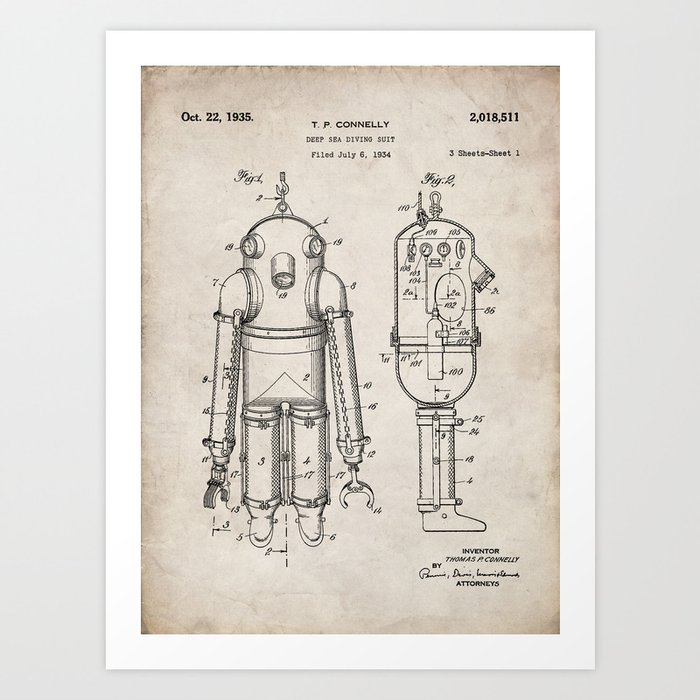This image features a rectangular poster with a light brown background and a white border, depicting a detailed mechanical drawing of a deep-sea diving suit invented by Thomas P. Connelly. The poster is divided into front and side views of the humanoid robotic suit, which has cylindrical arms and legs, two pipe-like eyes, a nose, and various labeled sections. Text at the top reads, "Oct 22, 1935, T. P. Connelly, Deep Sea Diving Suit, Filed July 6, 1934, 2,018,511, 3 sheets, sheet 1." At the bottom right, the text reads, "Inventor Thomas P. Connelly," along with his signature and the word "attorneys." The overall background of the image is light gray.